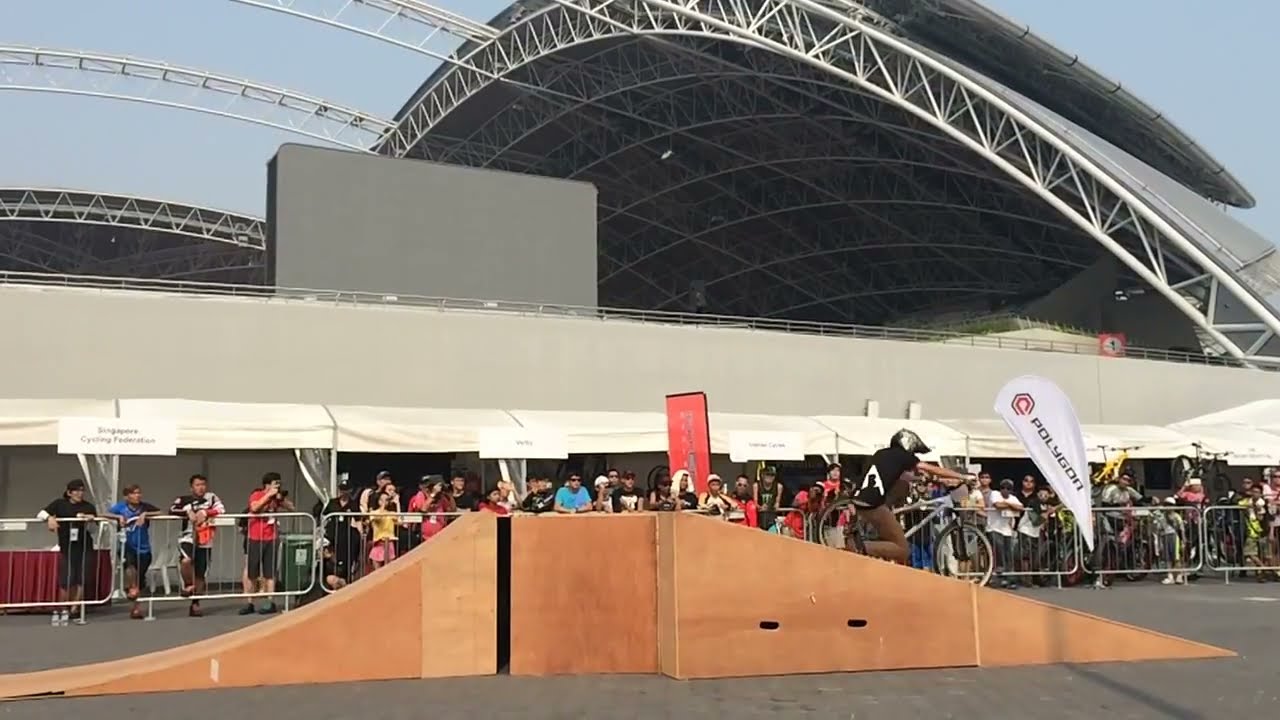In the foreground of the image, a BMX rider is captured on a wooden ramp. The ramp is located centrally at the bottom of the picture, and the biker, who wears a black shirt, khaki pants, and a silver helmet, appears poised after landing a jump, with his feet touching the ground. To the right of the biker is a white flag that reads "Polygon" with an emblem. Surrounding the ramp, several spectators, including younger children, are gathered behind metal fences, indicative of a staged competition environment. The onlookers, some dressed for biking, lean on the barricades in rapt attention. The background features a large, arching stadium structure with a curvy metal roof that has an open area in the center, revealing the blue sky above. White arches resembling railings or fences are also visible, adding to the architectural complexity. The setting suggests a dynamic and temporary arrangement designed for the event.